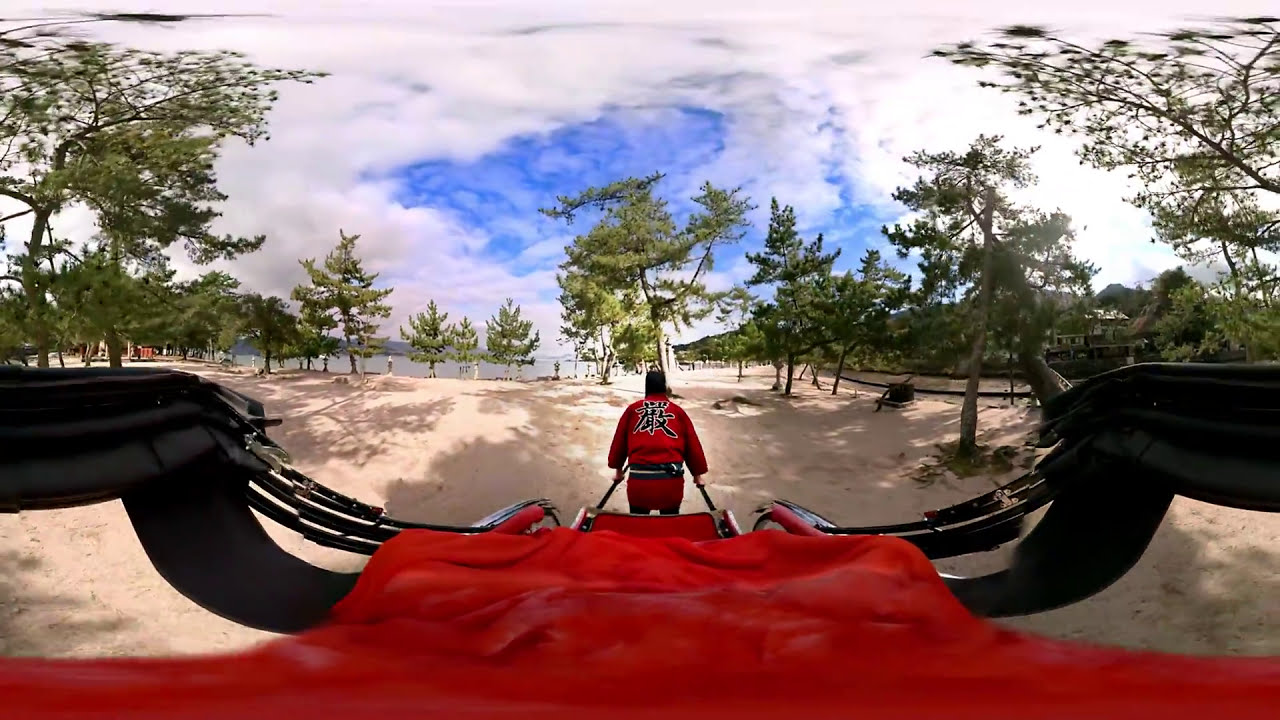In this photograph, we see the back of a man in a red uniform adorned with Chinese or Japanese writing. He appears to be pulling or guiding a red cart with black handles, suggesting some form of traditional taxi service. The cart, partially obscured and close to the camera, has a red top and seating with an odd distorted appearance, possibly due to panoramic stitching. The man is wearing a black headpiece and a black belt with a thin white stripe, and he’s walking on a light sandy path lined with green pine trees. Behind him, people stroll near a serene lake which merges into an ocean, while the bright blue sky, dotted with fluffy white clouds, stretches above. On the far right, there is a multi-level building nestled among the trees, enhancing the tranquil, picturesque scenery that resembles a park or coastal area in Japan.